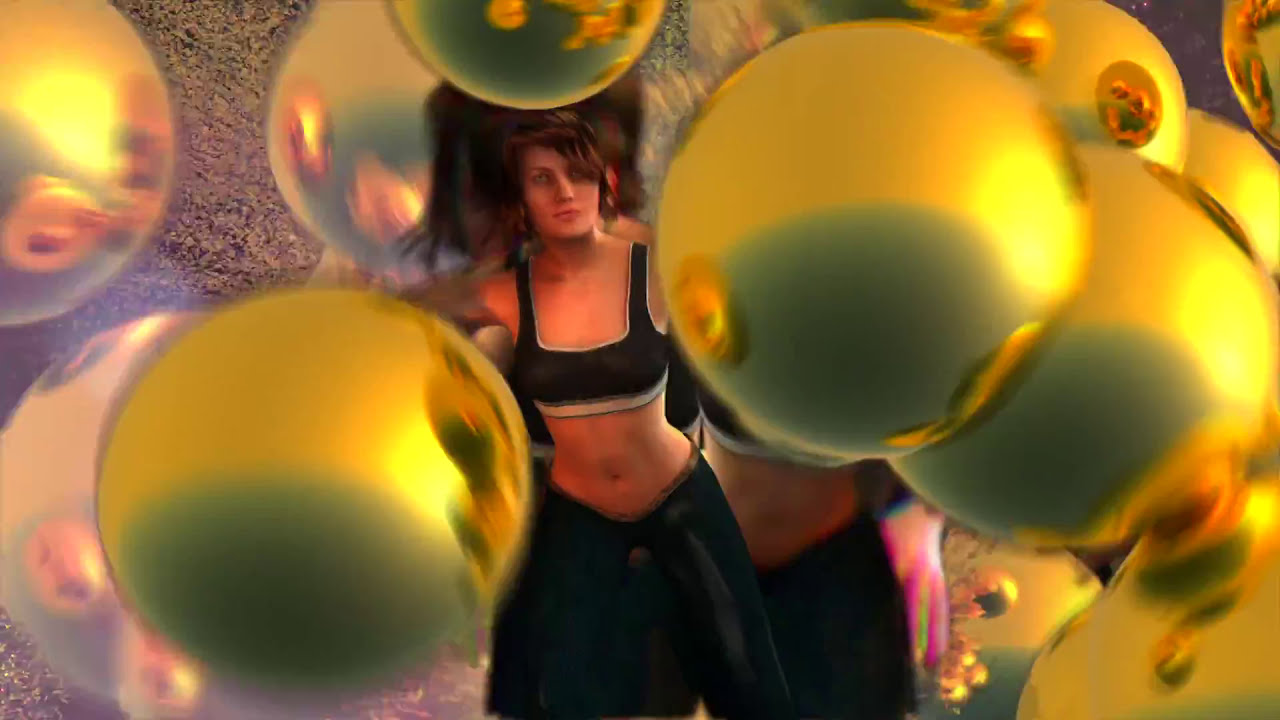In the center of the image, there is a female character with dark brown hair styled in bangs, pulled back, and a piercing, almost robotic gaze. She is wearing a black sports bra and tight black pants that sit low on her waist, revealing her belly button and toned midriff. The setting is almost surreal, adorned with numerous shiny, gold-colored balls and some pinkish-gray ones floating in the air against a light, granite-toned background. It appears the same woman is mirrored on her right, partially obscured by the golden orbs. The atmosphere evokes a sense of confusion, with suggestions of an unusual or fantastical scenario that might resemble a party or rave, indicated by the bizarre decorations and the character's intense expression.